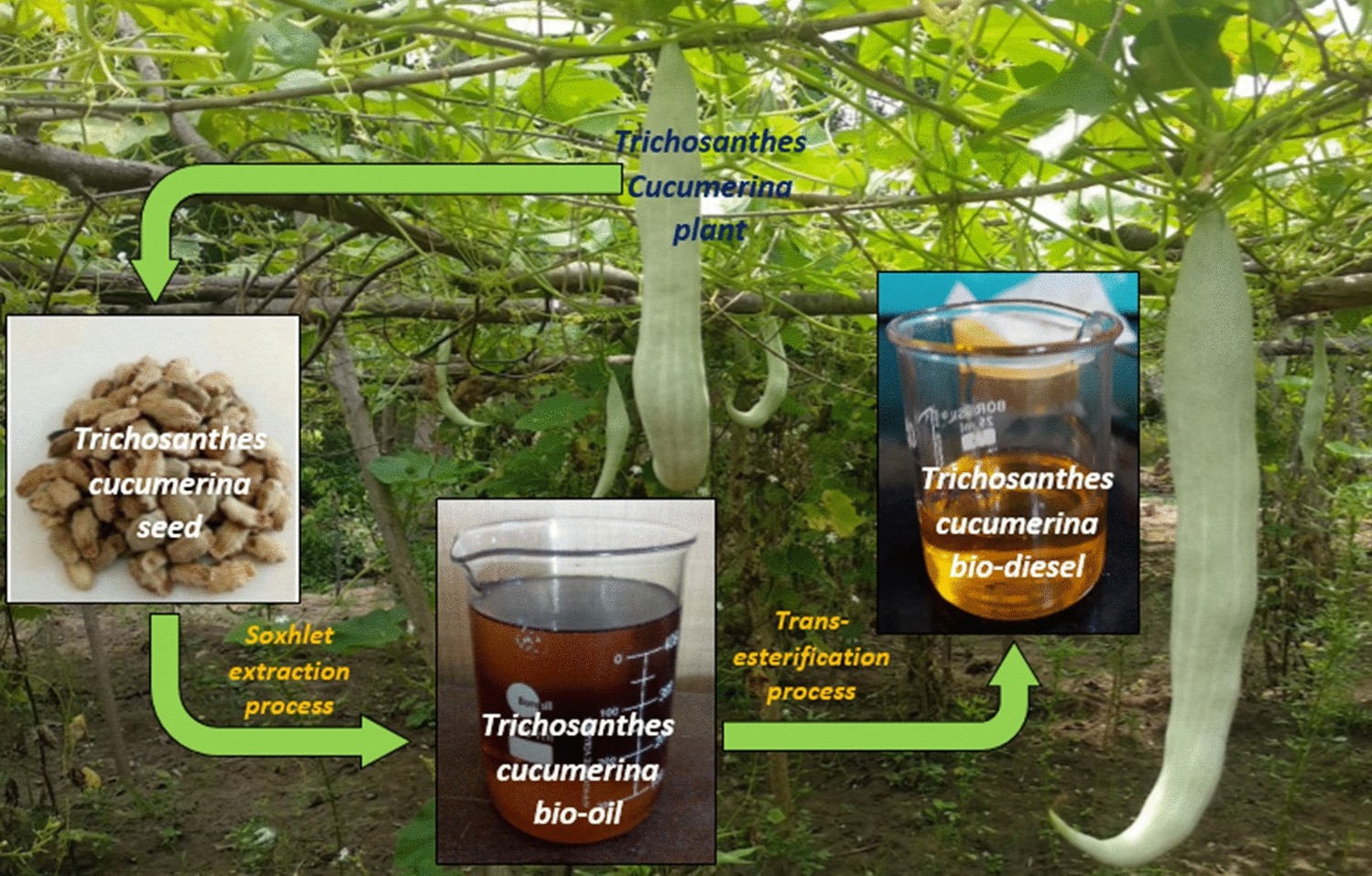This image illustrates the detailed process cycle of extracting bio-oil and biodiesel from the seeds of the *Trichosanthes cucumerina* plant.

At the top of the image, there's a photograph showcasing the *Trichosanthes cucumerina* plant, commonly known for producing cucumber-like fruits. The photograph captures the vines with numerous hanging cucumbers, providing a visual reference to the plant in question.

Proceeding to the right, the process is delineated with clear, labeled steps. Starting from the bottom left, there's an image depicting the *Trichosanthes cucumerina* seeds, which serve as the initial raw material for the extraction process. Next, the Soxhlet extraction process is illustrated. This scientific method involves using the seeds to obtain Trichosanthes Cucumerina bio-oil, represented by a beaker containing a dark liquid. 

Further along, we see another beaker filled with a lighter, oil-like liquid, labeled as *Trichosanthes cucumerina* biodiesel, indicating a refined product from the initial bio-oil. This step highlights the transition from raw bio-oil to biodiesel, suitable for fuel use.

Throughout the image, photographs of larger cucumbers are interspersed as background visuals, emphasizing the plant source continuously. The cycle ultimately showcases the journey of the *Trichosanthes cucumerina* seeds from their raw form through various processing stages to produce bio-oil and biodiesel, encapsulating the entire extraction pathway in a comprehensive and visually detailed manner.